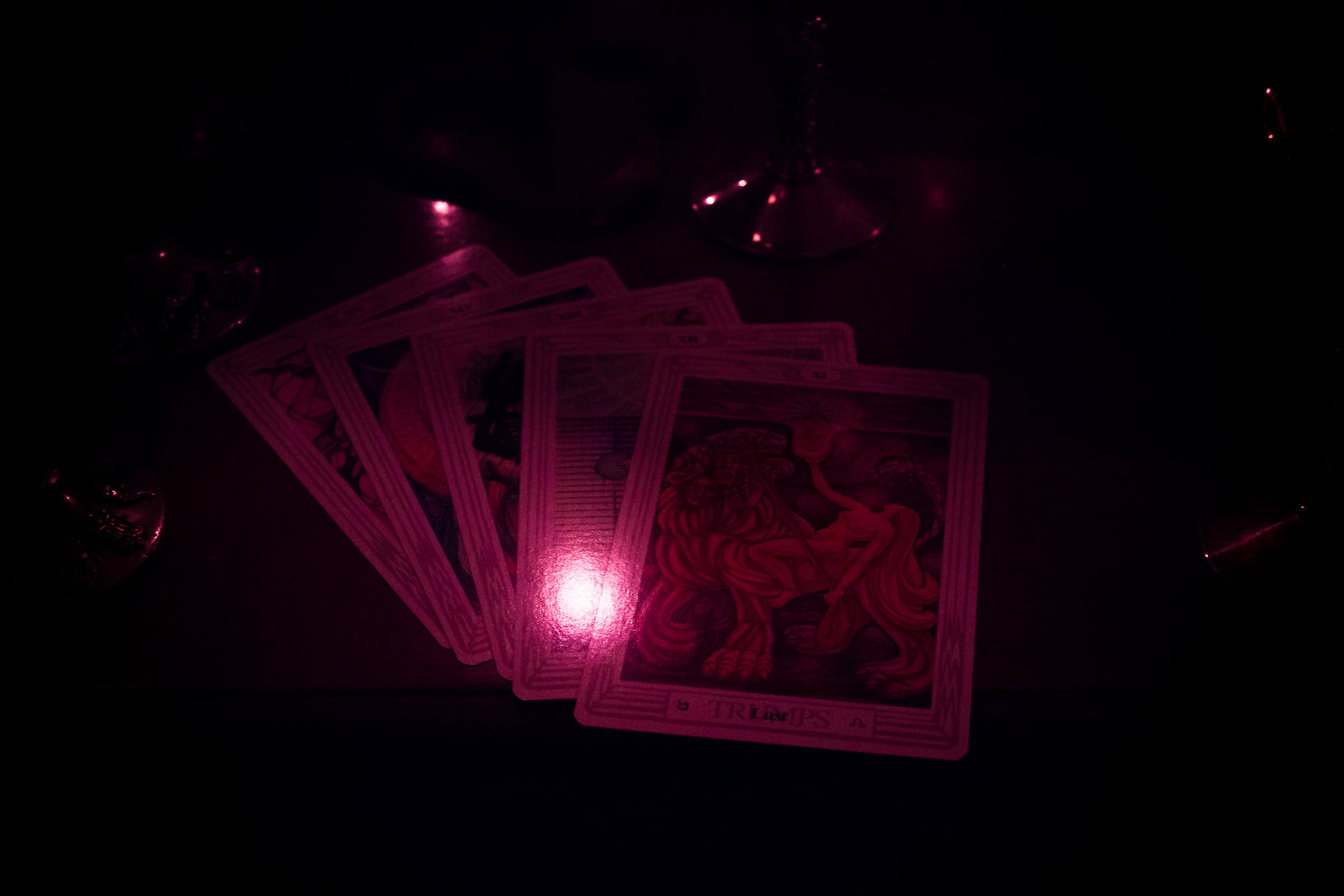In this dimly lit photograph, we see five playing cards positioned centrally on a table. The cards are arranged in a cascading spread, but their specific brand remains indistinguishable. The primary card in focus features a striking design with a purple outline. The bottom of this card bears the word "Trumps" inscribed in purplish-red lettering. The artwork on the card depicts a mythical creature: a topless woman, merging with an animalistic form. Her gaze is cast upward, hair cascading down, while her right arm appears to be pulling on something indistinct. The creature she is integrated with possesses noticeable legs and a face, blending human and beastly elements.

The remaining four cards are partially obscured, with one card particularly overexposed due to excessive light, rendering its details unclear. The photograph's dark ambiance makes it challenging to discern other background elements, but faint flashes of light streak across the top, adding a mysterious aura to the image.